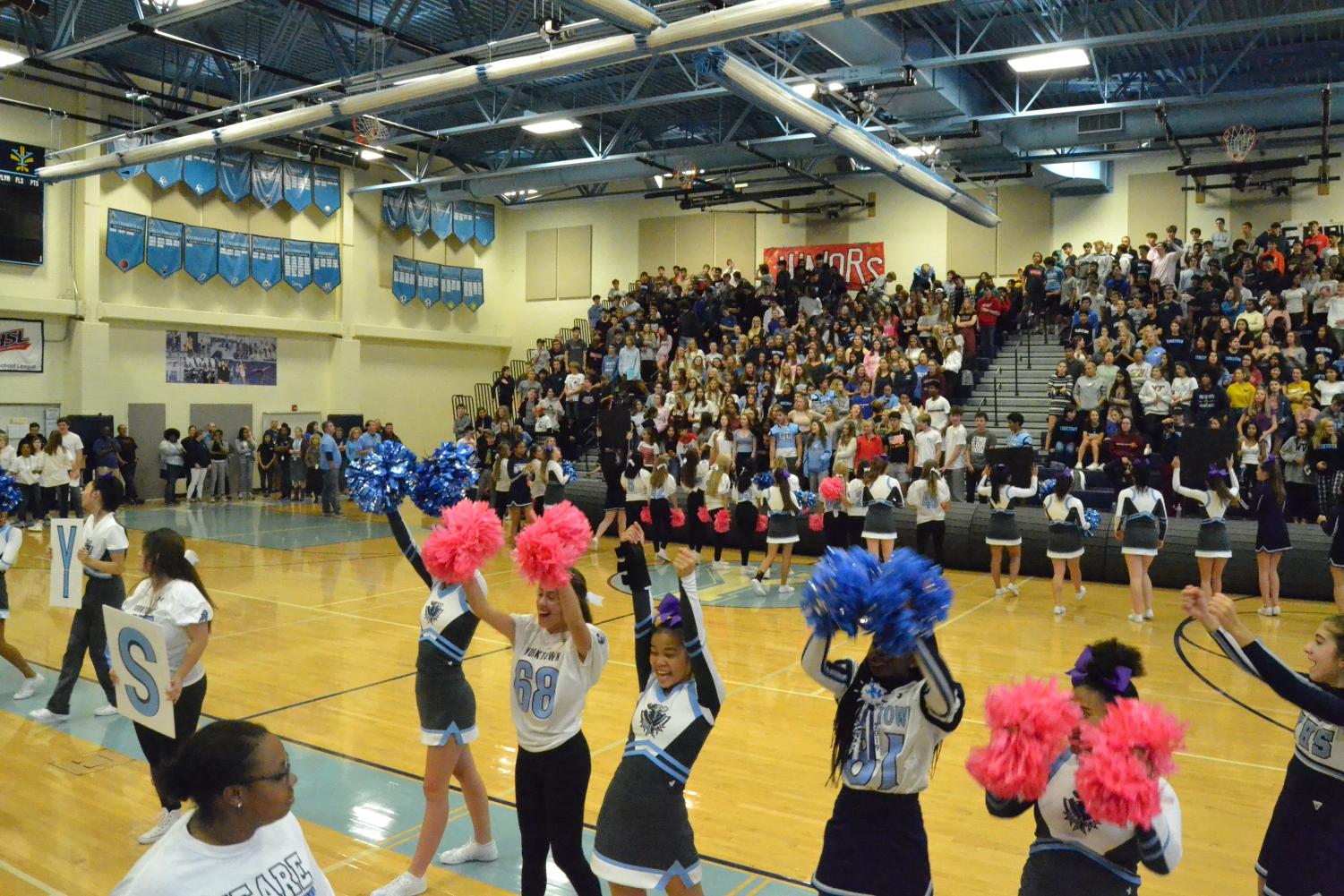This detailed image captures an energetic scene inside a large high school gymnasium during what appears to be a pep rally or a pre-game performance. The gymnasium ceiling features blue rafters, HVAC lights, and other equipment. The bleachers in the background are almost completely full, with some spectators standing in the back. In the foreground, a row of young cheerleaders in blue, white, and light blue uniforms are energetically dancing and holding up signs and pom-poms. Behind them on the basketball court, another row of cheerleaders mirrors their actions. One cheerleader stands out with pink pom-poms and a non-uniform white t-shirt and black pants. Various signs and decorations adorn the walls, although the text is mostly unreadable. On the sidelines, teachers and older individuals are observed conversing. The atmosphere in the gym is vibrant and lively, indicative of a well-attended school event.